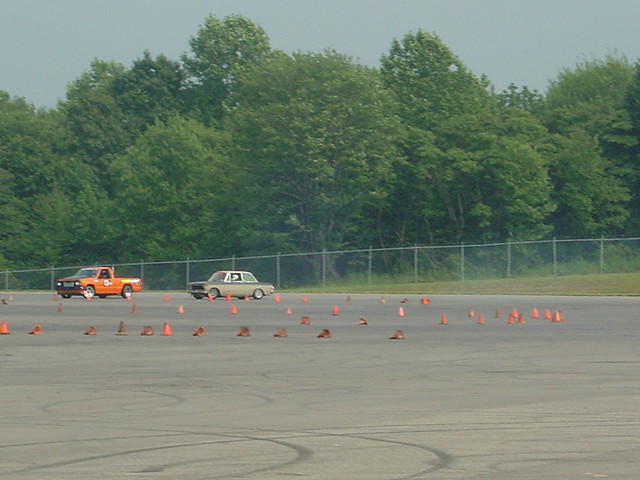In this hazy outdoor photograph, a large, mostly empty paved lot is depicted, encircled by a continuous gray metal chain-link fence. The expansive flat surface is dotted with numerous orange traffic cones, some of which lie toppled, alongside various skid marks that mar the pavement. Positioned within this setup are two distinct vehicles: an orange pickup truck adorned with logos, suggesting a racing or testing event, and a greenish-brown sedan, driven by a helmeted individual. The backdrop features a grassy field that transitions seamlessly into a lush, forested tree line characterized by a mixture of dark and light green foliage. Overhead, the sky is overcast with gray clouds, further contributing to the overall ambiance of the scene.